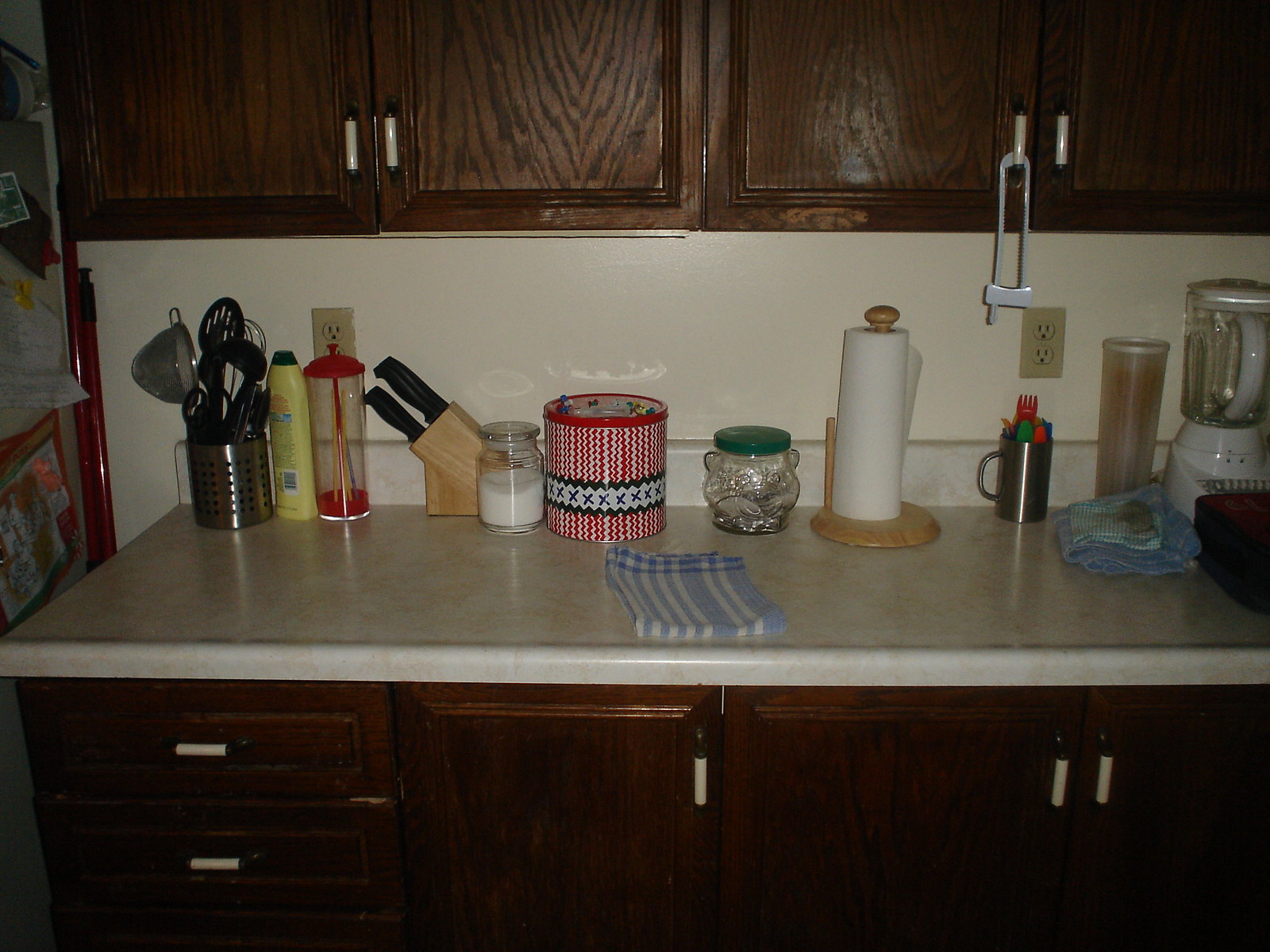On the white marble-like countertop, there is a silver tin holding an assortment of utensils and spatulas. Nearby, a light brown knife block, filled with sleek black knives, stands ready for use. A large, decorative cookie tin adds a touch of charm to the scene. Adjacent to this, a brown paper towel holder with a white paper towel roll sits conveniently within reach. A blue and white striped kitchen towel is neatly laid out, adding a pop of color to the setup. Off to the far right, a pristine white blender is partially visible, completing the organized kitchen space.